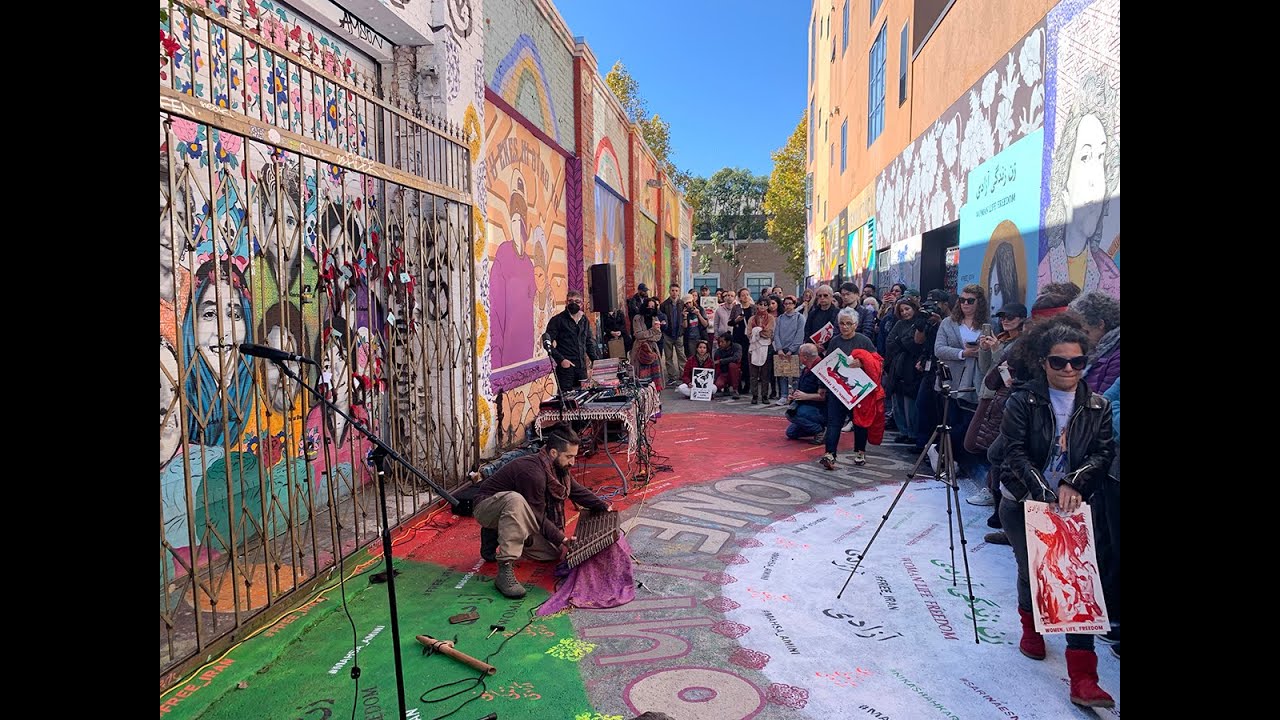The vibrant outdoor scene is set in an alleyway between two buildings, each adorned with colorful murals predominantly featuring various people's faces and possibly some political slogans. The walls burst with bright hues, including a mural of a man in a long-sleeve shirt standing in front of musical keyboards and another showcasing people of different races smiling together. Below these murals, a man kneels, unwrapping musical instruments from a purple blanket, indicating preparations for a live performance. The alley floor is also painted, displaying an array of murals, one featuring a half-circle with green and red paint. A light beige fence or gate stands in the foreground, adding to the lively and festive atmosphere under the clear, bright blue sky. People milling around are either holding bags or posters, suggesting the anticipation of either a political rally or a concert.